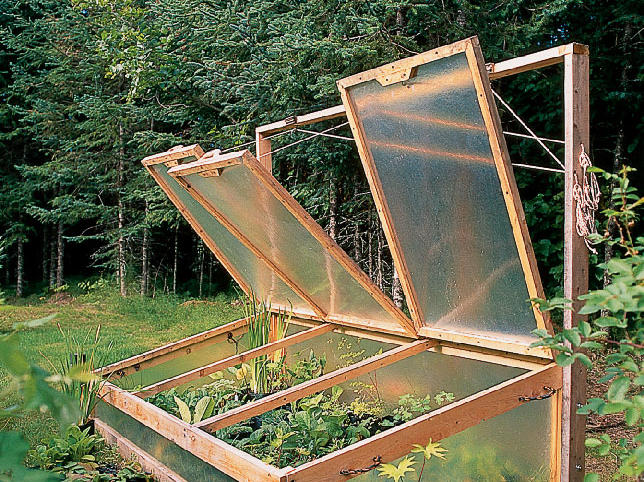The image depicts a detailed view of a small, rectangular greenhouse standing at approximately 5 to 10 feet across and 4 to 6 feet wide. Positioned on a grassy and dirt field, the greenhouse is seen from a 45-degree angle, highlighting its intricate design and construction. The greenhouse boasts glass or plexiglass walls and roofs made up of three individual lids. These lids are currently propped open with ropes attached to a rectangular wooden framework that rises behind the structure, allowing sunlight and air to nurture the vibrant plants within. Surrounding the greenhouse is a lush environment, with green conifer trees forming a dense backdrop, casting a dimly lit foundation. Additional foliage, including grass and bushes, frames the greenhouse in the foreground and to its sides, suggesting it is situated at the edge of a property bordering a verdant, impenetrable forest.